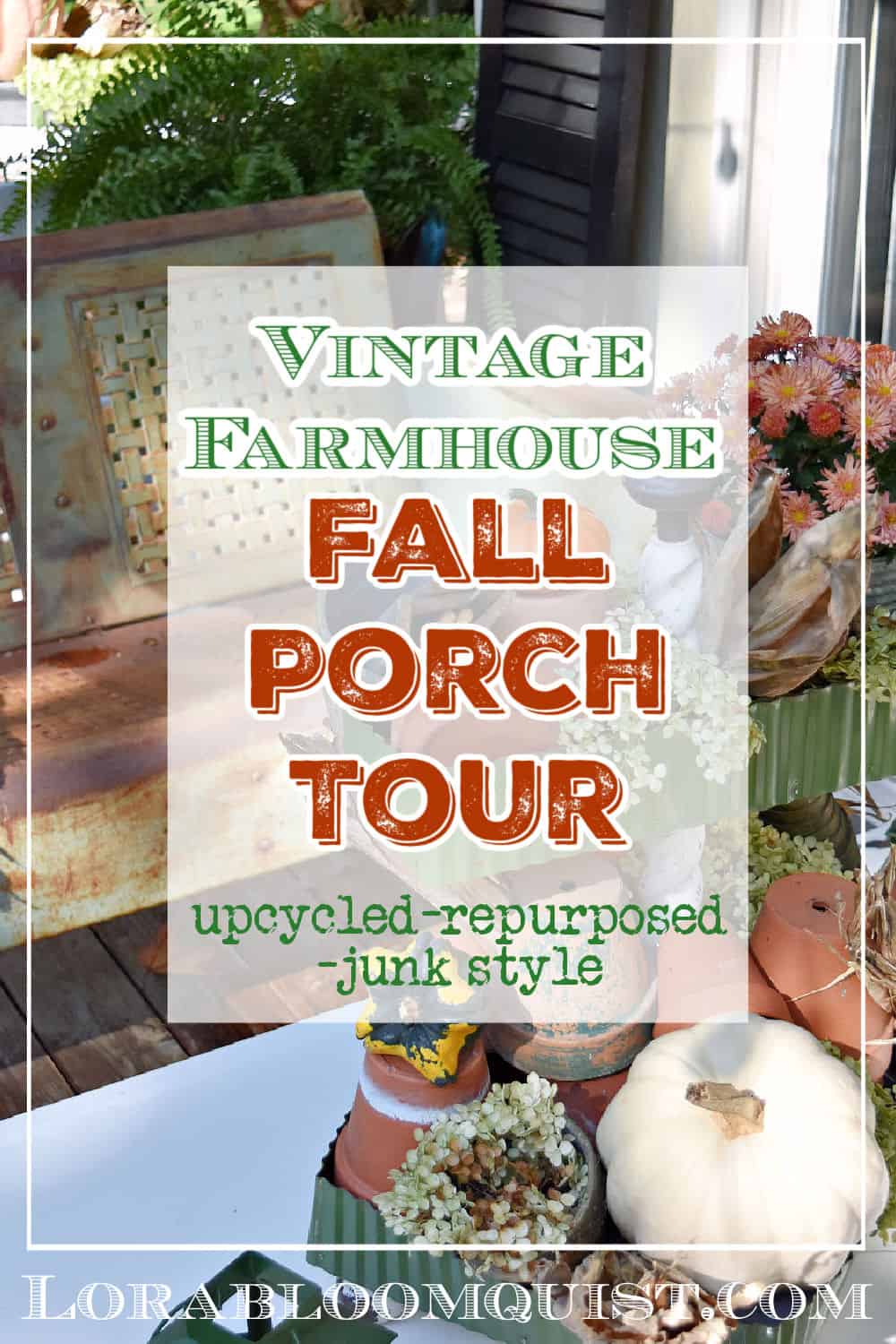The image appears to be a square book cover or magazine page featuring a beautifully decorated porch. The layout comprises an outer square with a white border, within which is a translucent white square containing text. This text, starting at the top in green and red fonts on a white background, reads: "Vintage Farmhouse Fall Porch Tour, Upcycled, Repurposed, Junk Style." The background image showcases a rustic porch adorned with various elements: a rustic bench, potted plants, a white pumpkin or gourd sitting on a white table, and a blue tray holding some of the plants. Behind the porch decor, the setting includes a house with black walls and a white door, where a green plant sits on the window sill with the window open. Additionally, pink flowers are also part of the decor. At the bottom of the image, in translucent text, is the website LauraBloomQuist.com. This precise arrangement suggests the cover promotes a decorating guide for a "Vintage Farmhouse Fall Porch Tour."